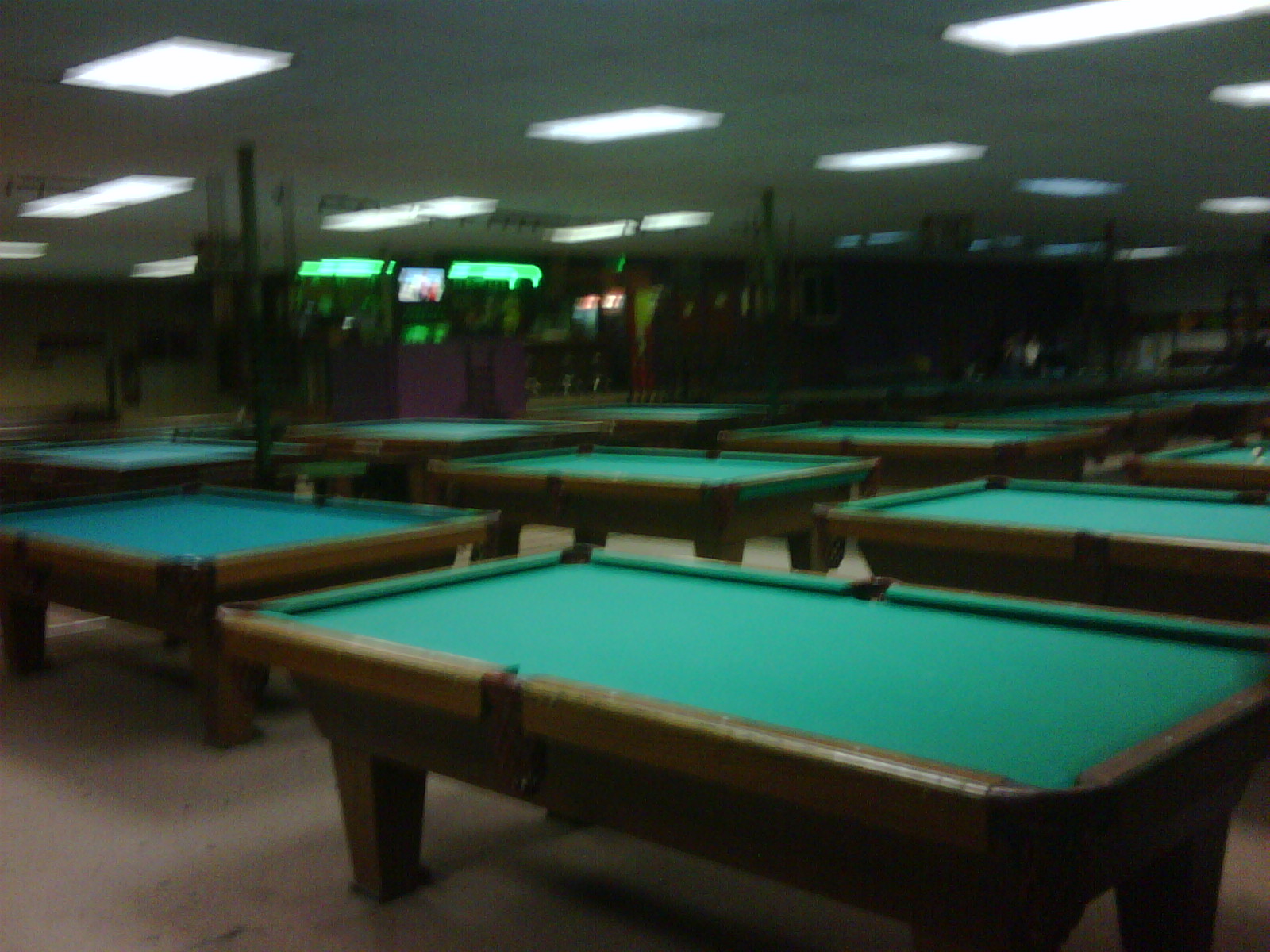This image captures an expansive, empty pool hall seen from a standing height perspective, with rows upon rows of identical pool tables stretching across the frame. The tables, framed in a combination of leather and wood, are predominantly covered in green felt, although a couple feature blue felt tops. These tables align in symmetrical rows, extending horizontally and at an angle, creating a visually pleasing repetition. Overhead, the white ceiling is punctuated by fluorescent lights, casting a even glow over the space. The background includes some neon signs, green signage, and what appears to be an elevated platform area that might house an arcade or a bar. The walls of the room have a purple hue, and the hard floor tiles reflect the room's ambient light. The atmosphere of the hall is quiet and still, as it is devoid of any people or equipment like pool balls or sticks.